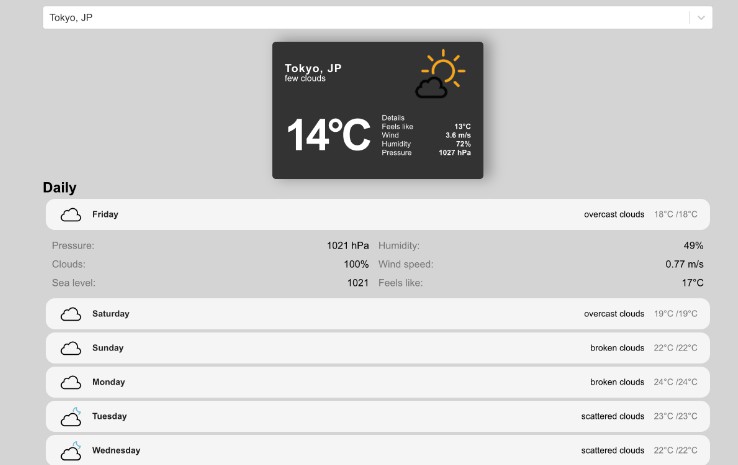A screenshot taken from a weather application displays detailed weather information for Tokyo, Japan. The background is gray, and at the top of the screen slightly inset from both the left and right edges, there is a search bar. On the left side of the search bar, "Tokyo JP" is written in black text, indicating the location, with a dropdown arrow on the right side of the bar for additional options.

Below the search bar, there's a central black box with white text. It reiterates "Tokyo JP," followed by descriptions of the weather conditions. Written in large text is "14°C," with a surrounding degree symbol indicating the temperature. Accompanying the temperature is an icon of a yellow sun partially covered by a black cloud, symbolizing cloudy weather with some sun. 

Underneath the current temperature, the detailed weather conditions are listed: 
- "Feels like 13°C" gives a more accurate sense of the perceived temperature.
- "Wind: 3.6 m/s" indicates the wind speed.
- "Humidity: 72%" shows the moisture level in the air.
- "Pressure: 1072 hPa" indicates the atmospheric pressure.

A daily forecast section covers the weather from Friday through Wednesday, with temperatures ranging from a low of 18°C to a high of 24°C. The screen also includes additional metrics such as the current pressure, humidity, and cloud coverage, which is at 100%. The wind speed is listed again, and sea level pressure is shown at "1021 hPa." The text mentions that it currently feels like 17°C, reflecting the perceived temperature at that moment.

Overall, the image captures a comprehensive snapshot of the weather details, providing clear and detailed information about the current and upcoming weather conditions in Tokyo, Japan.